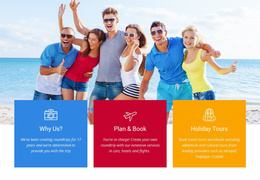This website screenshot showcases an inviting outdoor photograph of a group of young adults standing in a line, either holding on to one another or waving. The vibrant background features a breathtaking scene of turquoise water meeting a blue sky adorned with white clouds, with glimpses of white sand visible. Starting from the left, there is a young man wearing a white and blue shirt, giving a thumbs-up and sporting sunglasses. Next to him, a girl in a red tank top and short denim shorts is waving her arm, laughing, with her dark brown long hair flowing. To her right stands a tall man in a gray t-shirt, denim shorts, and sunglasses. Beside him is a young girl in a white t-shirt and blue and white shorts, with short brown hair and sunglasses. The lineup concludes with another young couple. Below the image, there are three colored informational boxes: the first blue box reads "Why Us?", the second red box says "Plan and Book" and features an airplane icon, followed by "Holiday Tours."